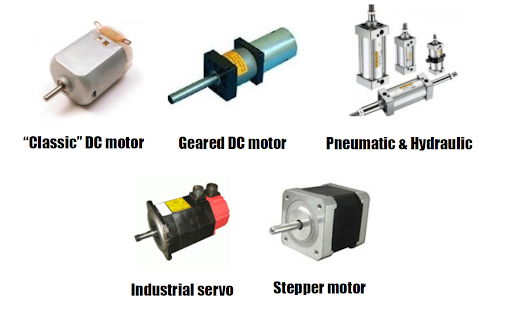The image presents five different types of small metallic objects, each a variation of motor or hydraulic components, arranged in a 3x2 grid with labels beneath each. From left to right, the top row includes a "Classic DC Motor" depicted as a small gray rectangular object with a metallic shaft protruding from the left side, a "Geared DC Motor" which is blue with a black plastic encasement and a central shaft emerging from it, and a "Pneumatic and Hydraulic" section showcasing four silver metallic cylindrical components with shafts, either upright or laid on a base. The bottom row features an "Industrial Servo," colored black with a red back piece, grayish shaft, and black buttons alongside yellow and white labels, and a "Stepper Motor," which looks like a slightly elongated cube with silver ends, a protruding shaft, and four holes for screws, marked by its gray metallic body with black elements.